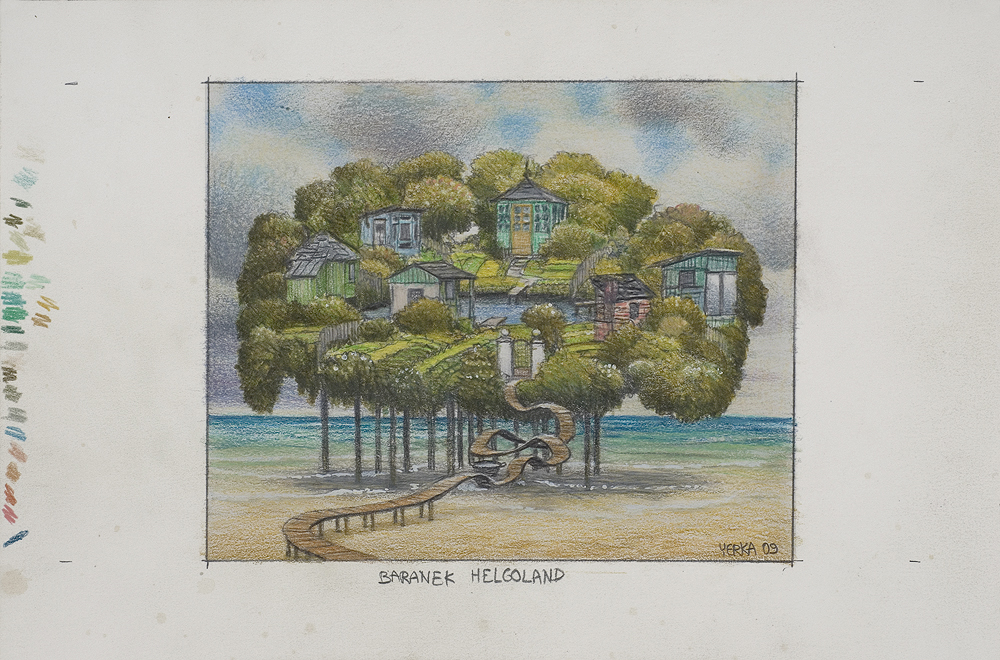The artwork features a surreal treehouse village set against a beige backdrop. Central to the piece is a framed square image set within a larger white rectangle. On the left side of the frame, colored pencil test marks in hues of blue, green, and red add an artistic touch. Below this inset image, the words "Berenak Helgoland" are sketched. Inside the square, "Y-E-R-K-A O-9" is prominently written. The scene depicts an imaginative wooden boardwalk that swirls and ascends to a treehouse-like village perched on tall stilts. This whimsical pathway leads up to a cluster of seven quaint, saltbox-style houses nestled in the canopy. The houses are small, painted blue and green, and appear to float above a sandy beach with turquoise waters that fade into a rich green. The sky painted in the backdrop showcases beautiful, puffy clouds with shades of purple and blue. The entire composition evokes a dreamlike atmosphere, blending elements of nature with fantastical architecture.